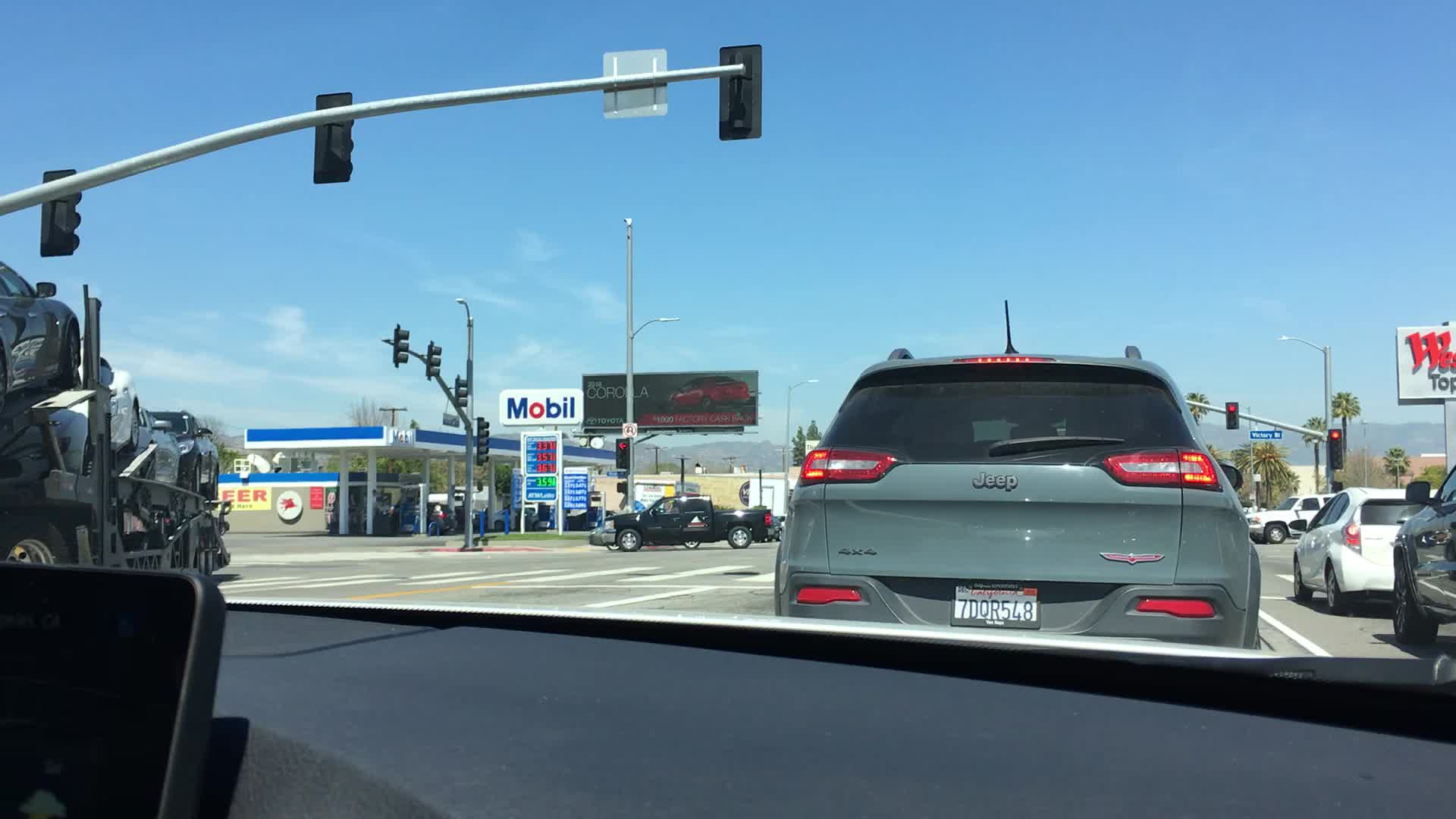The image depicts the interior of a vehicle's passenger compartment with a focus on its dark-colored dashboard. Dominating the dashboard, there's a prominent display screen embedded within a dark housing; the screen is off, appearing as a sleek black glass surface, likely meant for computer readouts. 

Through the vehicle's windshield, a green sport utility Jeep with a white license plate is visible directly in front. To the right of the Jeep, a small white car sits at a crosswalk beneath a red traffic light on a steel pole. Additionally, another traffic light, housed in a black casing with the red light illuminated, is positioned at the street corner.

On the left side of the frame, a blue and white overhang from a gas station marked with a "Mobil" sign featuring blue and red print sits prominently. In the vicinity, a light blue pickup truck is captured mid-turn at the intersection. The scene unfolds under a bright midday sky with minimal cloud cover.